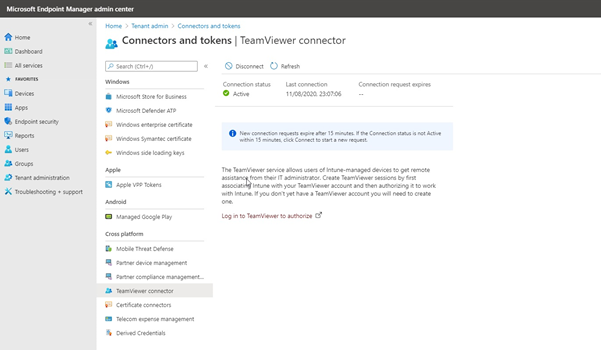Here's a cleaned-up and detailed caption for the image:

---

The image showcases a detailed screenshot of the Microsoft Endpoint Manager Admin Center interface. At the top, there is a slim black bar running horizontally across the width of the screen. Inside this bar, small white text reads "Microsoft Endpoint Manager Admin Center."

On the left side, there is a vertical blue sidebar. In the upper right corner of the sidebar, there is an 'X' or 'arrow' symbol, likely for navigation purposes. Below this, various icons and menu items are listed: 
- A blue house icon labeled "Home"
- "Dashboard"
- "All Services"
- "Favorites"
- "Devices"
- "Apps"
- "Endpoint Security"
- "Reports"
- "Users"
- "Groups"
- "Templates"
- "Admin"
- "Administration"
- "Troubleshooting + Support"

The main content area, occupying the right side of the screen, has a white background. At the top, there are blue-tabbed headings: "Home," "Tenant Admin," "Connectors," and "Tokens." Beneath this, two blue outline icons of people and a title in black text read "Connectors and Tokens." 

Below this title is a white search bar labeled "Search." To the right of the search bar, black text options for "Disconnect" and "Refresh" are available.

Further down on the left side under the search bar, there are additional menu items listed:
- "Windows"
- "Microsoft Store for Business"
- "Microsoft Defender"
- Items related to Windows, Apple, and Android
- "Cross Platform"

At the bottom of the sidebar, there is an indication of an active connection with details: "Active connection on 11-06-2020 at 23:07:06."

---

This caption provides a clear and comprehensive description of the various elements and layout visible in the screenshot.